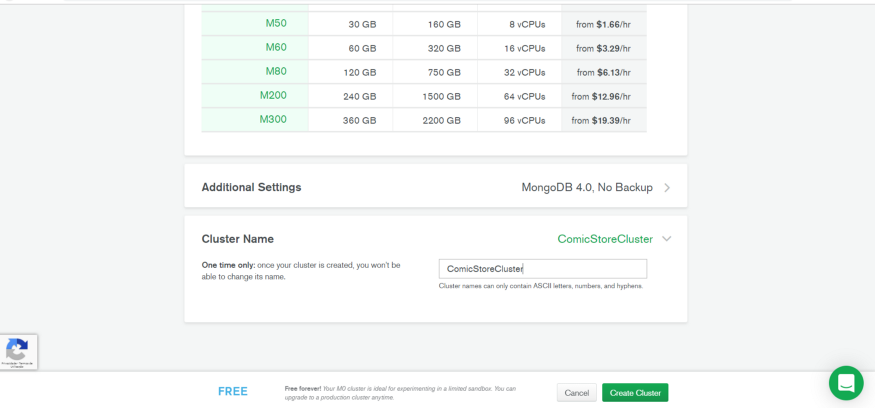This image depicts a detailed configuration page for setting up a Comic Store Cluster in a cloud service dashboard. At the top, the page features five dropdown entries arranged horizontally. Vertically, the chart lists various machine types and their associated specifications in individual boxes:

- **M5 Cluster**
  - **RAM**: 30 GB
  - **Storage**: 160 GB
  - **vCPUs**: 4 (166 per hour)
  
- **M60 Cluster**
  - **RAM**: 60 GB
  - **Storage**: 320 GB
  - **vCPUs**: 8, 16 (329 per hour)
  
- **M80 Cluster**
  - **RAM**: 120 GB
  - **Storage**: 750 GB
  - **vCPUs**: 32 (613 per hour)
  
- **M200 Cluster**
  - **RAM**: 240 GB
  - **Storage**: 1,500 GB
  - **vCPUs**: 64 (1296 per hour)
  
- **M300 Cluster**
  - **RAM**: 360 GB
  - **Storage**: 2,200 GB
  - **vCPUs**: 96 (1939 per hour)

Below these specifications, there is an "Additional Settings" section categorizing the configuration for MongoDB 4.0 without backup. A right-facing arrow suggests more options are available.

Further down, a box labeled "Cluster Name" emphasizes that the cluster name can only be set once, instructing that it is a one-time entry which cannot be altered later. To the right of this box, the default name "Comic Store Cluster" appears with a dropdown arrow, allowing for selection from pre-existing options. Inside a search box labeled "Comic Store Cluster," the cursor blinks at the end of the query.

The bottom of the page features a note indicating the service is "Free Forever," alongside a "Cancel" button and a prominent "Create Cluster" button. There's also an interactive chat bot available for assistance on the right-hand side of the page.